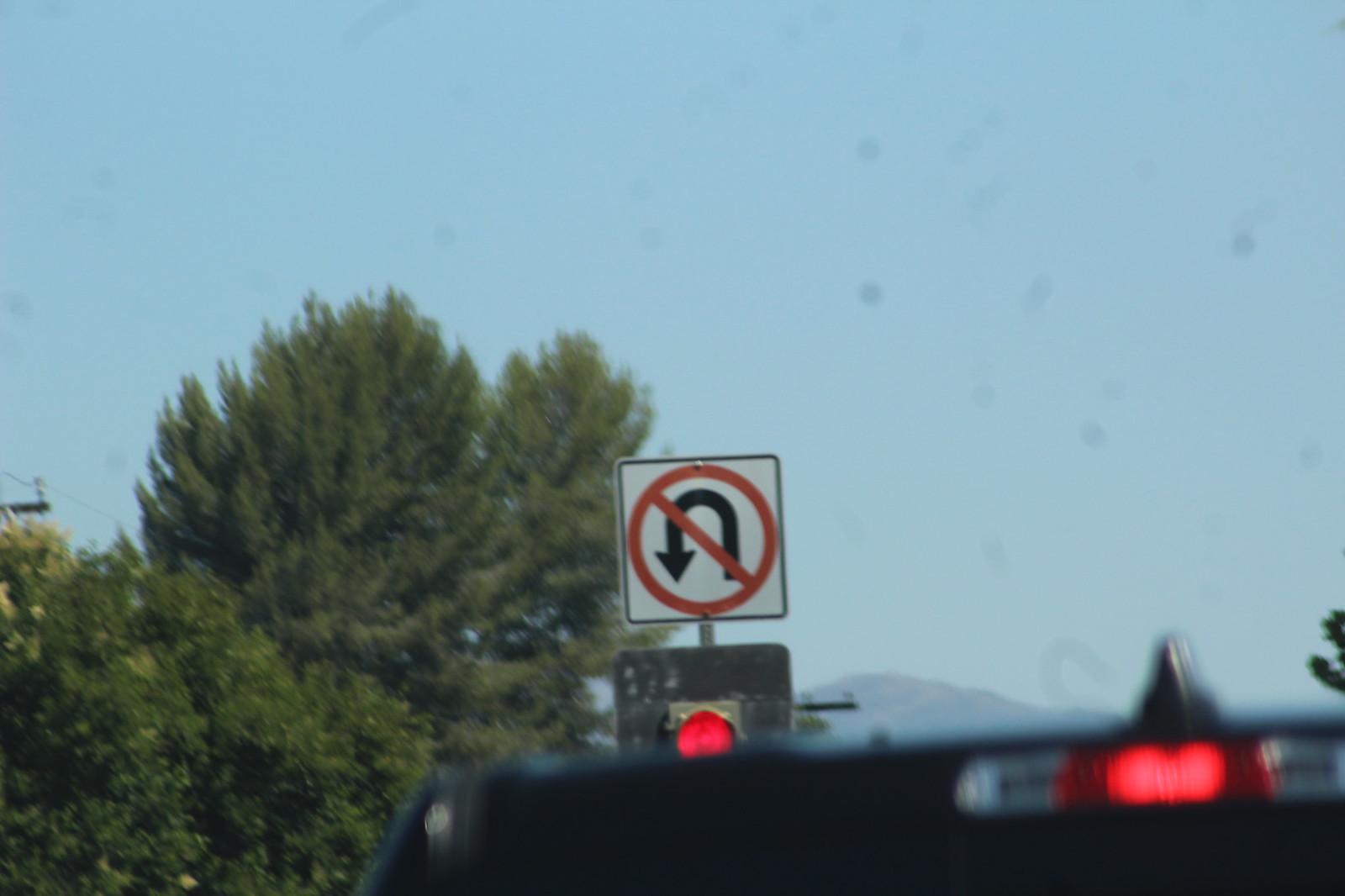A photograph captures a street sign as its central focal point against a medium light blue sky. The image appears to have been taken through a slightly dirty windshield, evidenced by small spots on the right-hand side and top of the photo. In the left background, two deciduous trees with lush green leaves frame the scene. The bottom portion of the image shows what may be the front interior of a vehicle, including part of a black dashboard and a red indicator light on the right side.

Dominating the center is a prominent street sign with a white background. The sign features a red circle encompassing an inverted U with a downward-pointing arrow on its left, crossed out by a red slash, signifying 'No U-turn.' Beneath this sign, the upper section of a gray traffic light is visible, with its topmost light illuminated in red.